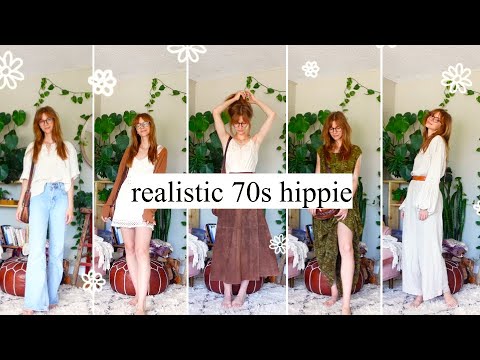The horizontally rectangular image features a series of five vertically rectangular photographs of a tall, red-haired woman depicted in different 70s-inspired outfits. The overall photo is framed with thick black borders on the top and bottom. Each vertical section is separated by thin white lines, and there are outlined images of white flowers in the background. A central white banner divides the images, bearing the text "Realistic 70s Hippie."

1. In the far-left image, the woman has her hair down, wears glasses, a white shirt tucked into blue jeans, and carries a brown purse over her right shoulder.
   
2. The second image showcases her in a white sundress paired with a brown cardigan, still with her glasses on.

3. At the center, the woman has her hair put up, dons a white top over a long, reddish-pink skirt and carries a purse.

4. The fourth image features her in a sleeveless long green dress, looking down at something in her hands.

5. Finally, on the far right, she is wearing a full-length white gown with an orange belt, posing in a room that has a white wall, green vine leaves, and various accessories.